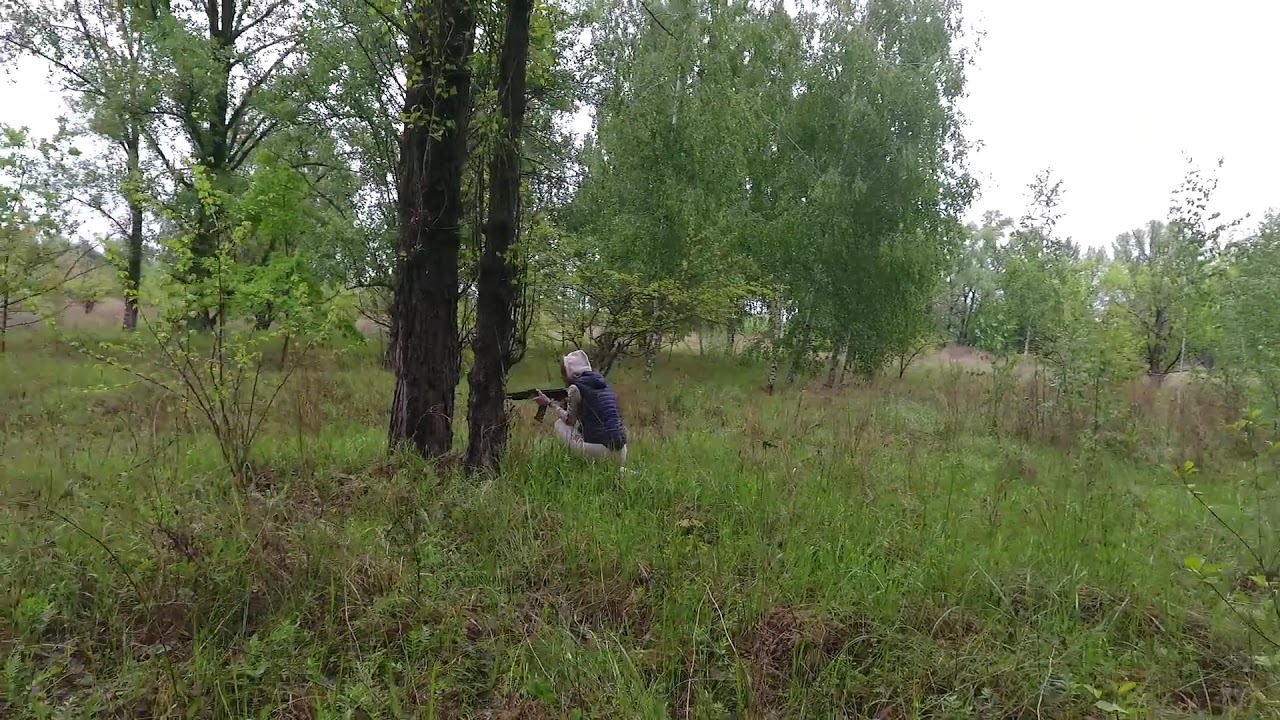In this outdoor photograph, a person is depicted crouching amidst tall, unkempt grass and shrubbery, partially concealed behind three vine-covered, brown tree trunks. The individual is dressed in gray pants, a white hoodie with the hood up, and a blue puffer vest, which also has a hood, though it is not being worn. The person cradles an assault rifle, possibly an AK-47, with a visible magazine, aimed towards the left side of the image, suggesting a vigilant stance. The scene is set in a lightly forested area with a mix of tall green and brown grass and scattered bushes with short, leafy branches. In the distance, a field and additional trees are visible under a gray, overcast sky, and the sun is not shining. There are no other people in the image.